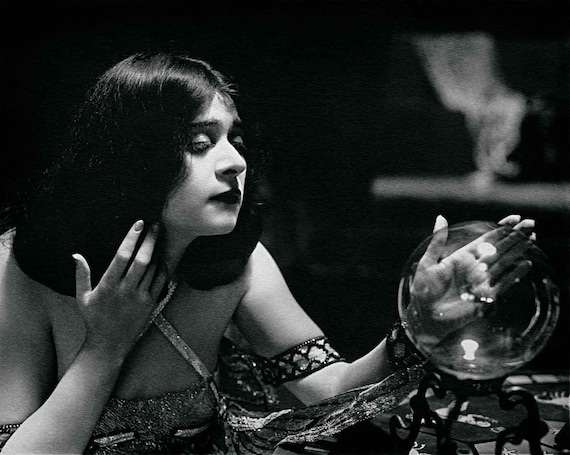In this striking black-and-white photograph, a woman with neatly trimmed, shoulder-length black hair styled in a shapely, fluffy bob is depicted as a fortune teller or gypsy. She is positioned on the left side of the image, wearing dark makeup and lipstick, which accentuates her forlorn expression. Her attire includes a sleeveless or revealing top with decorative straps crisscrossing her chest, and a unique ornamental band wrapped around her upper arm. The woman's left hand hovers beside a luminous crystal ball, which rests on a small pedestal clad in cloth and possibly adorned with engravings. Her right hand, with pointed nails, is partially visible near her neck. In the background, a wisp of smoke ascends gracefully in the top right corner, adding a mystical atmosphere to the scene.